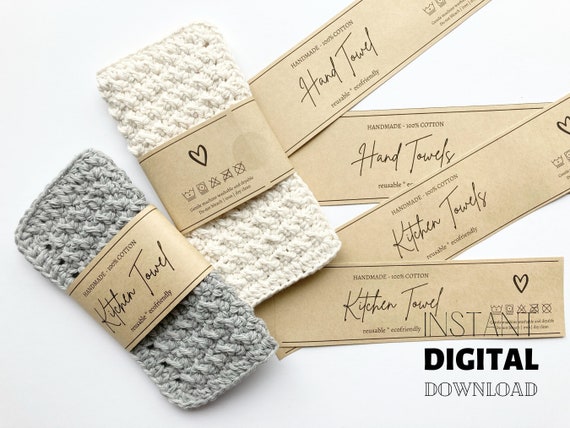The image is a product advertisement showcasing two kitchen towels, one grey on the left and one white on the right, both intricately made with cross stitching. Set against a white-greyish backdrop, resembling a table, these towels are packaged with a central paper label. The label prominently reads "handmade, 100% cotton, kitchen towel, reusable, eco-friendly," with an illustrated heart and washing icons on the reverse side. Additional labels, mirroring the same text and symbols, are scattered to the right. The lower right corner of the image features the watermark "instant digital download," suggesting the product is available for immediate online purchase.